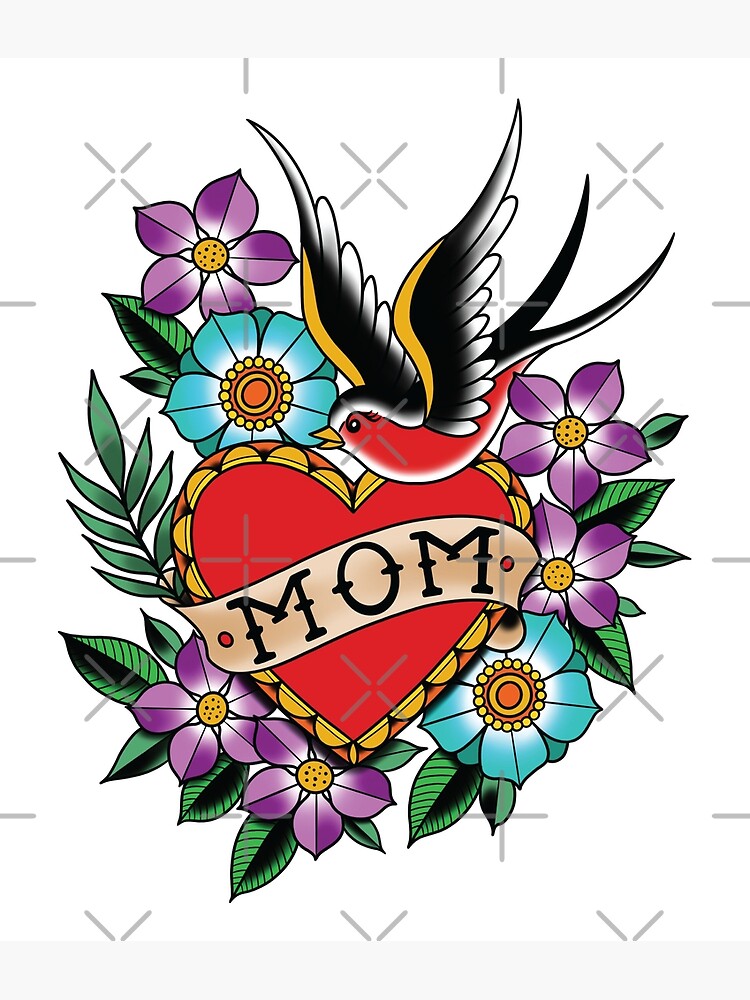The cartoon-like image, possibly designed as a vibrant tattoo template, features a red heart with a lattice edging of gold and orange at its center. The heart is adorned with a tan, diagonal banner that reads "MOM" in black, capital letters. Above the heart, a bird with a red breast is in flight, its beak pointing to the left and its tail feathers to the right. The bird's wings are black with yellow edges on top and white edgings below. Surrounding the heart and bird are an array of teal and purple flowers, specifically five purple flowers—their placement includes clusters at the bottom left, to the right-hand side, and one at the top left. There are also blue flowers, one positioned at the top left and another at the bottom right of the heart, each with circular yellow and orange centers. Interspersed among the flowers are green leaves, including one that resembles a fern. The entire scene is set against a white background detailed with light gray plus and minus signs, possibly for sizing purposes.